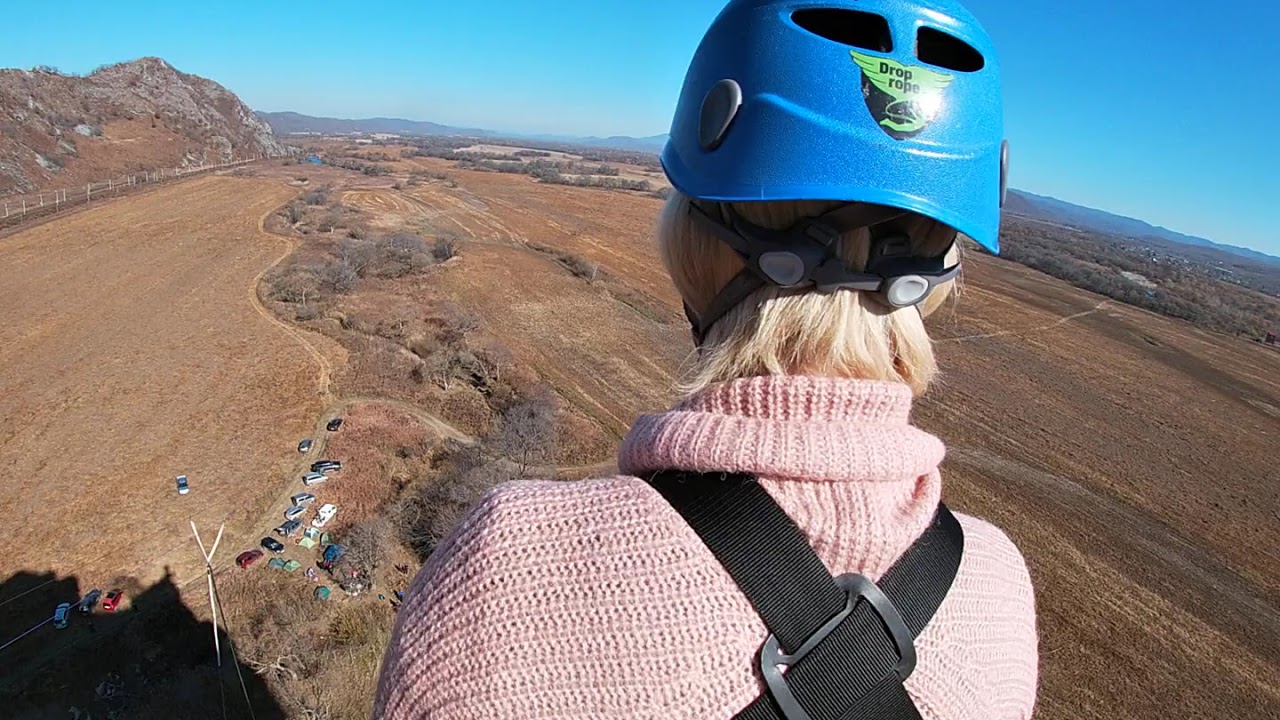The image captures the back of a person who appears to be on the verge of a bungee jump, seen from mid-back to the top of their head. The individual is clad in a pink knit sweater, with a black harness that crisscrosses over their back. Their short blonde hair is tucked into a blue helmet adorned with a green logo and the black text "drop rope." The scene suggests a high-altitude setting as the ground below appears far away. The landscape is a patchwork of reddish and brown fields, with leafless, brown-colored trees visible through their branches. On the left, large reddish rock hills rise against the horizon, while dark, hilled mountainous areas stretch into the distance on the right. The bright blue sky above transitions from a deeper blue at the top to a lighter hue near the horizon. Far below, you can discern very small, color-varied cars parked along a roadway, and a windmill standing amidst the fields, reinforcing the vast height from which the person is preparing to jump.